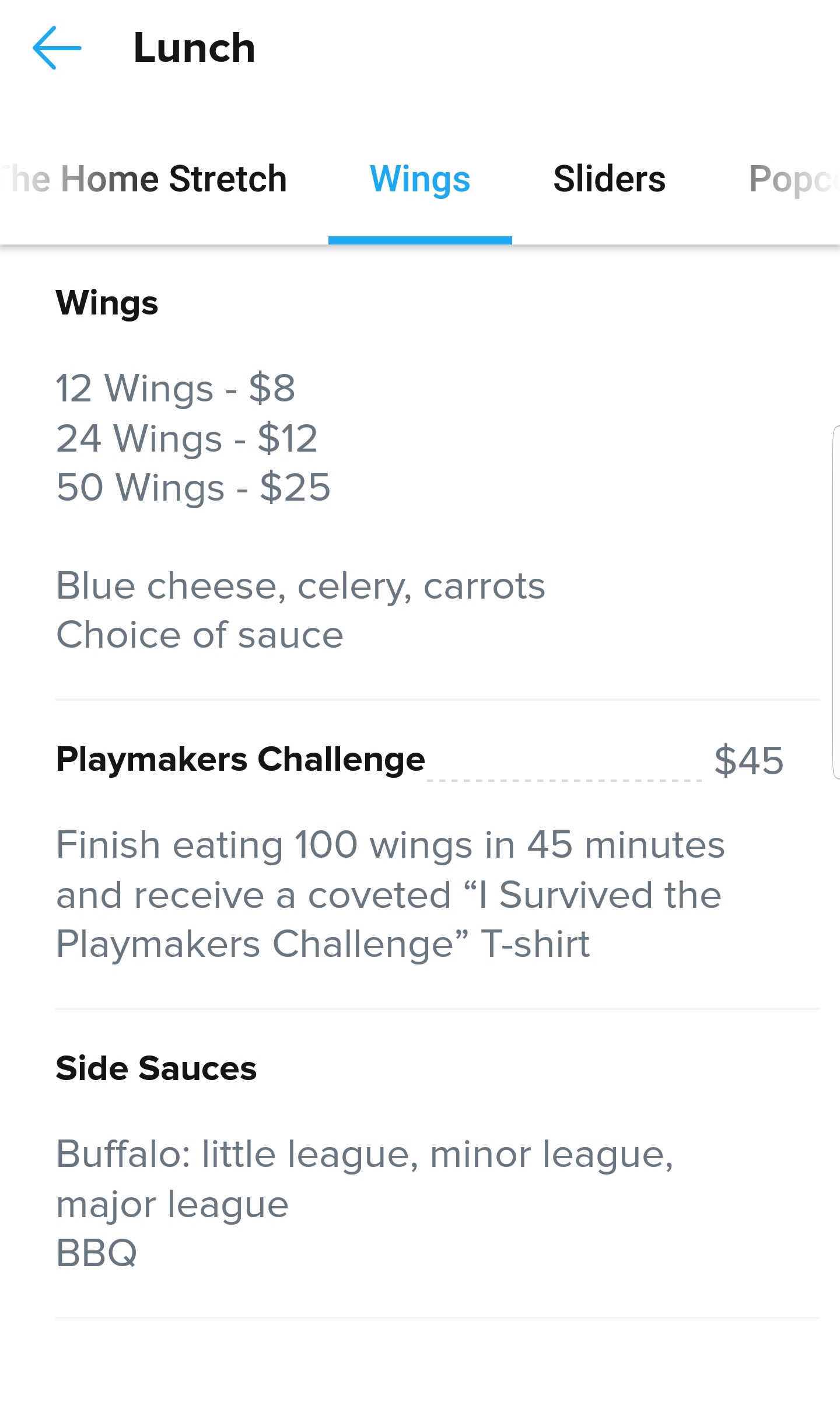This image depicts a page from a restaurant menu with a focus on their wing offerings. The background is predominantly white. In the top left corner, there is a black text reading "Lunch" accompanied by a blue back arrow to its left. Below, a horizontal menu bar features several tabs. The selected tab is "Wings," highlighted in blue, while other tabs, such as "The Home Stretch," "Sliders," and another partially visible tab possibly labeled "Popcorn," are also present.

The main content under the "Wings" tab lists the various wing options and prices:
- 12 wings for $8
- 24 wings for $12
- 50 wings for $25

Each portion includes blue cheese, celery, carrots, and a choice of sauce. Additionally, there is a special promotion called the "Playmakers Challenge," priced at $45. It challenges diners to finish 100 wings in 45 minutes, with the reward of an exclusive "I Survived the Playmakers Challenge" t-shirt upon completion.

At the bottom, the menu lists the available side sauces, which include Buffalo, Little League, Minor League, Major League, and Barbecue.

This image captures the restaurant's wing offerings and the accompanying sauces available for a personalized dining experience.